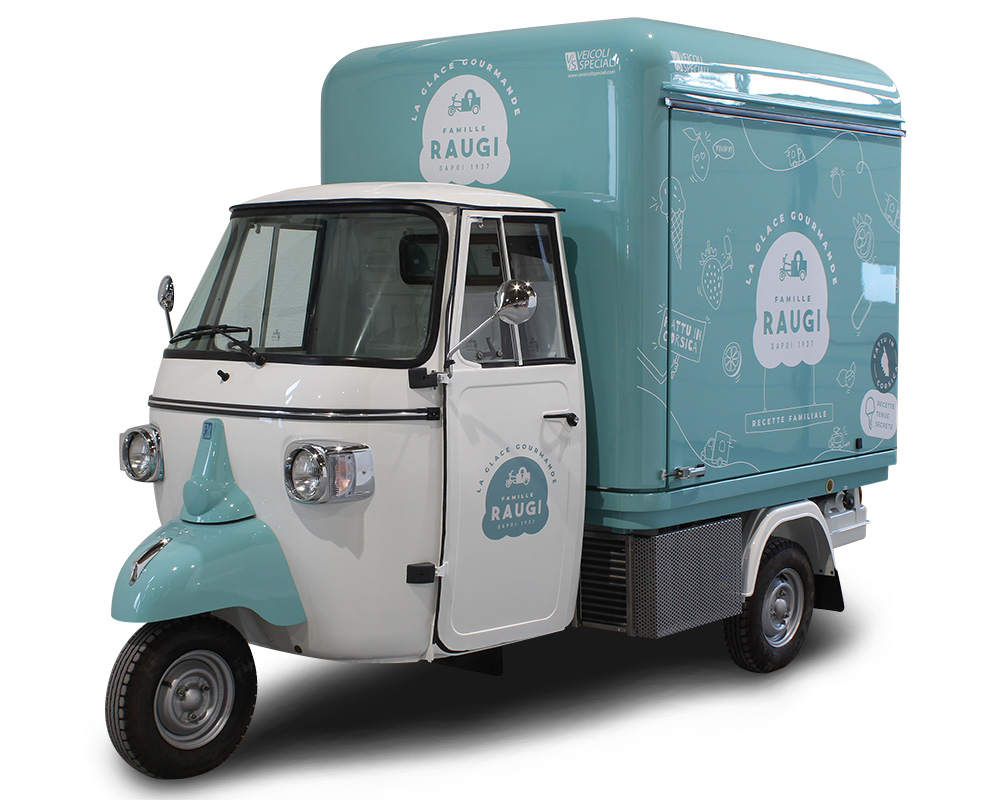This is a detailed color photograph of a vintage-styled, three-wheeled ice cream or gelato delivery vehicle, set against a completely white background. The cab of the truck is predominantly white with chrome headlights, complemented by a bright turquoise front section over one wheel. The back portion, also turquoise, features a large cooler-type storage unit and two black wheels, with only one wheel visible. The truck, oriented to the left, is adorned with white illustrations, including an image of a strawberry holding an ice cream cone, a lemon, and a drawing of the truck driving along a hill. Prominently displayed are the names "La Glace Gourmand," "Famille Rougie," and "Recette Familiere," suggesting a French origin. The vehicle embodies a nostalgic 1960s aesthetic but appears brand new, clean, and shiny.